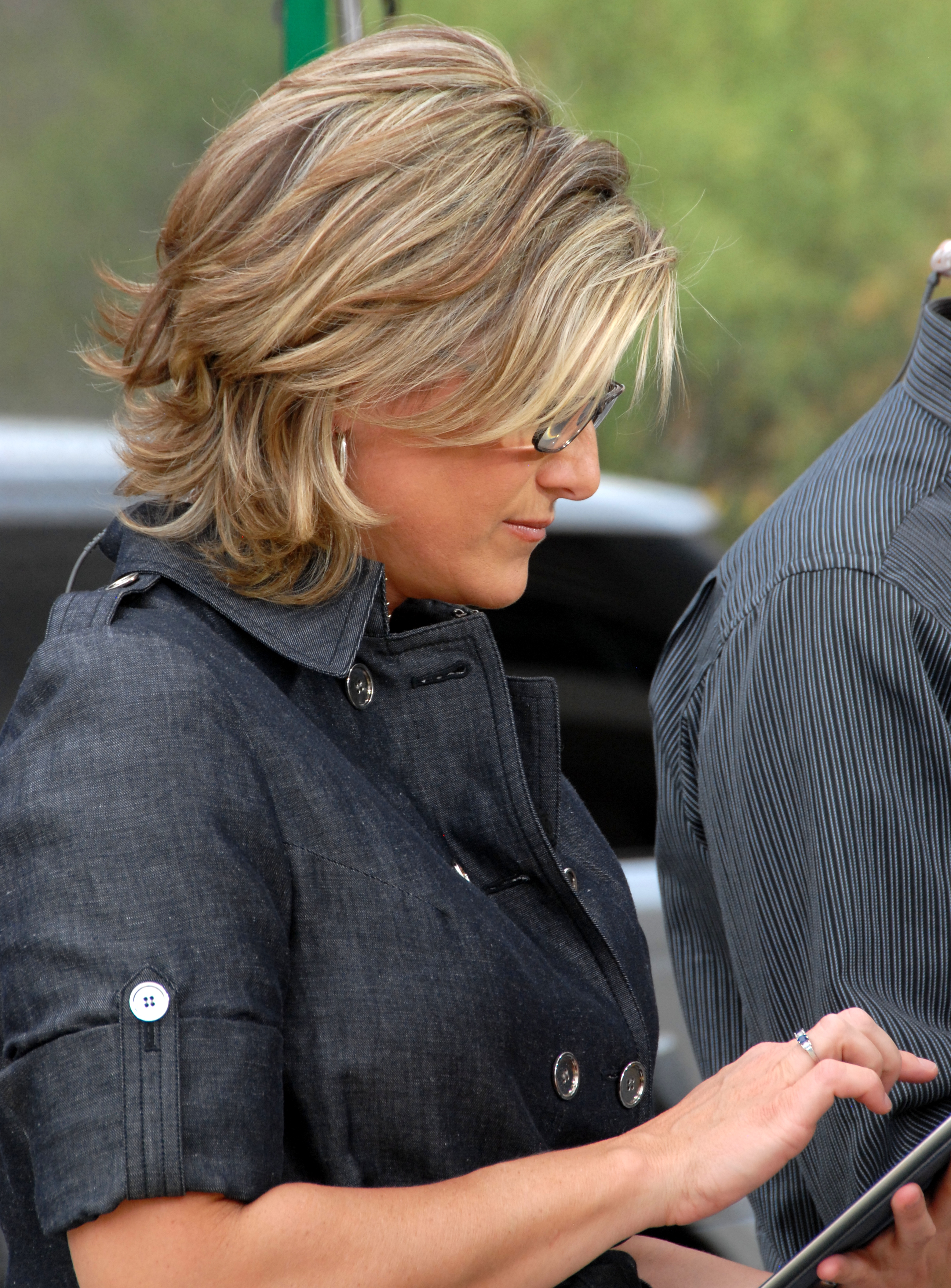In this detailed photograph, a woman with shoulder-length blonde hair and black-rimmed glasses is captured in a side profile as she interacts with her smartphone. She is intently looking down at the device in her right hand, her index finger pointed towards the screen, indicating active engagement. Her right hand also sports a striking silver ring with two white diamonds and a blue gem nestled in between. Adorning her ears are noticeable hoop earrings that complement her look.

She is dressed in a stylish denim coat featuring multiple silver buttons, with her left hand subtly supporting the bottom of the smartphone. The out-of-focus background reveals a lush expanse of green vegetation, adding a natural, serene touch to the scene. Additionally, to the right, the shoulder of another person clad in a gray shirt can be faintly seen, along with a white vehicle with black windows, contributing an urban context to the photograph.